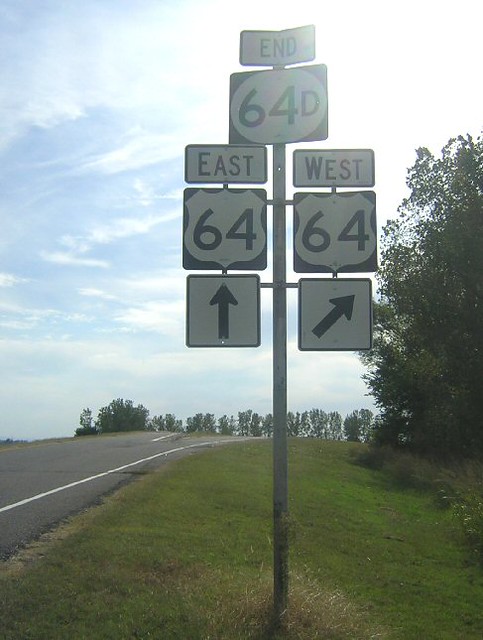In this image of the outdoors, we see a blue sky filled with wispy white clouds and a bright white sun glowing in the top right corner. Below, a grassy field stretches out, dotted with green trees on both the right, middle back, and left sides. The scene captures a highway with the road extending to the left and a silver pole prominently positioned almost in the center of the image. The pole supports multiple signs: at the top, it reads "END 64D" while on the left side, a sign indicates "EAST 64" with a black arrow pointing straight ahead. On the right side, another sign directs "WEST 64" with an arrow pointing to the right. The quality of the photo suggests it was taken with an older camera or phone, adding a nostalgic touch to this crisp and detailed outdoor scene. The road appears to go over a hill, potentially merging off ahead where the sign indicates.